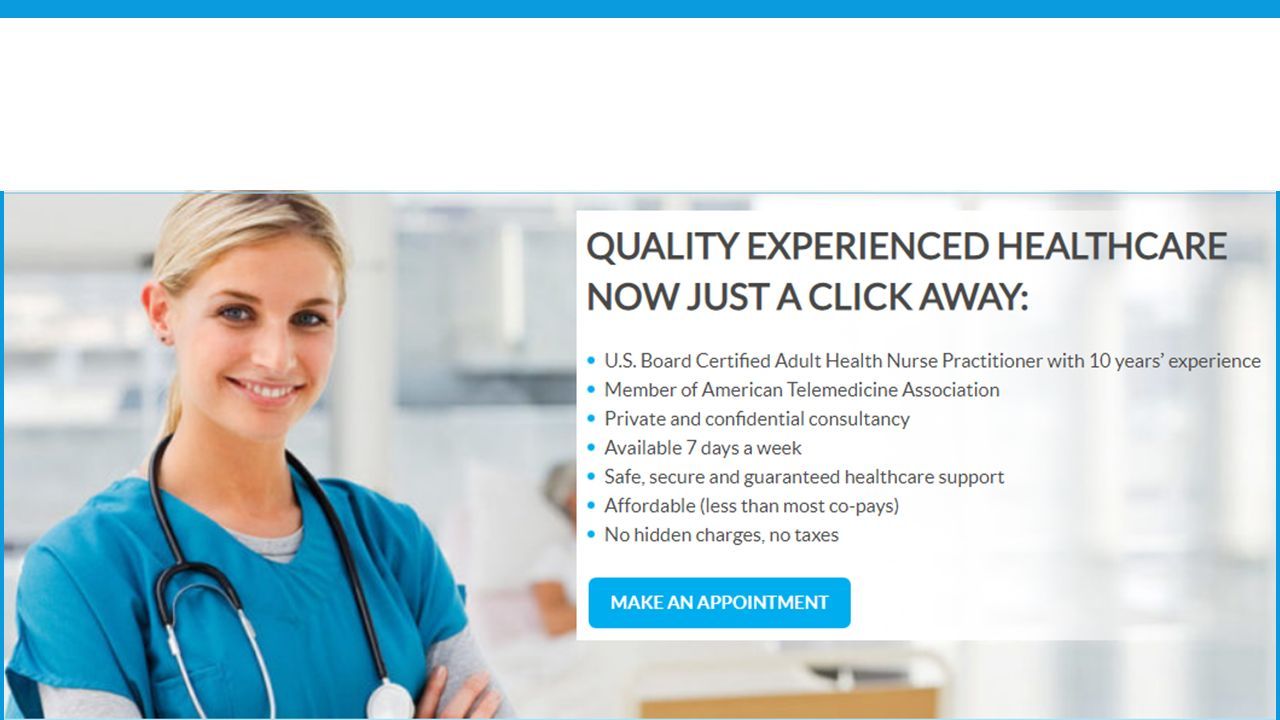This is a detailed caption for a screenshot of a health care website advertisement. 

In the background, there is a photograph of a young female nurse with blonde hair, dressed in blue scrubs with a light gray undershirt. She has a stethoscope around her neck and is smiling while standing with her arms folded. To the right of the image, a white, semi-transparent box overlays the photograph. The box, marked with a faint watermark, contains text in bold, black, all-caps font at the top that reads "QUALITY EXPERIENCED HEALTH CARE." Below, in smaller black font, the description continues with "Now just a click away." Underneath, there are seven bullet points detailing the service offerings: a nurse practitioner with 10 years of experience, various qualifications listed, availability 7 days a week, safe and secure services, absence of hidden charges, and no taxes. This advertisement highlights the key features of the health care services being promoted.